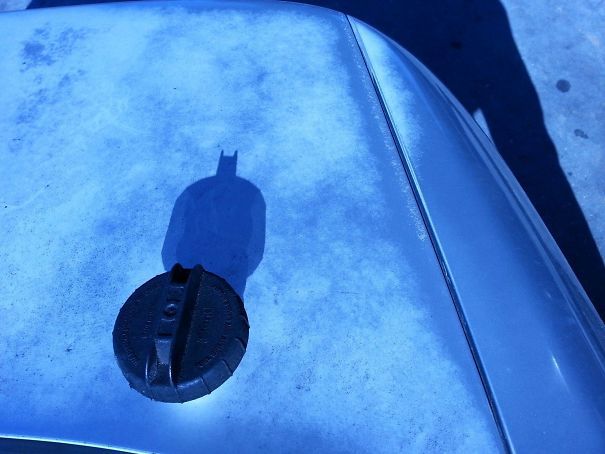A top-down view reveals the hood of a car, specifically the right side, rendered in a monochromatic purple hue. The paint is visibly faded, evident from the weather-worn texture on the surface. Bathed in sunlight, the hood casts distinct shadows. Notably, a large, black, round plastic cap sits prominently on the hood, its imposing form creating an intriguing shadow that mimics the iconic outline of Batman, the famed comic book superhero.